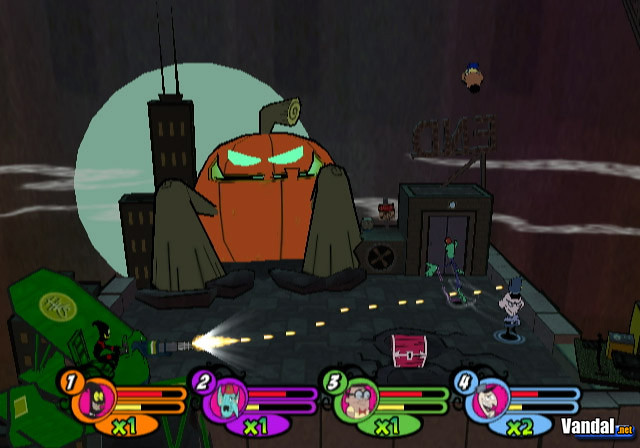The image depicts a dark, Halloween-themed, cartoonish mobile game scene filled with eerie details. A giant jack-o'-lantern with glowing eyes and a carved mouth featuring a tooth prominently looms in the background, blended with the night sky and a full moon. The jack-o'-lantern also appears to have arms, one extending towards a skyscraper. The scene is set on a series of rooftops, with a shadowy shed to the right, identifiable by its almost black appearance and a small green door. There is a red-topped building nestled between the jack-o'-lantern and the shed, amidst swirling white streaks in the sky that suggest clouds.

In the foreground, a trail crosses the lower half of the image, punctuated by an arrow of light. One character, seemingly about to enter an elevator, stands near a treasure chest on one rooftop, while another, dressed in a gray outfit and hat, exudes an evil demeanor. Overhead, a peculiar creature appears to be piloting a plane, possibly targeting the menacing figure below.

The bottom of the image features a game interface with four characters, each marked with distinctive colors and numbers—orange, purple, green, and blue—reflecting their health or power levels. The first character has a head with big round eyes, the second sports a blue head with red hair and an open mouth, the third is a bespectacled man, and the fourth is a peculiar small white head. The bottom right corner of the image is branded "vandal.net," hinting at the game's source or platform.